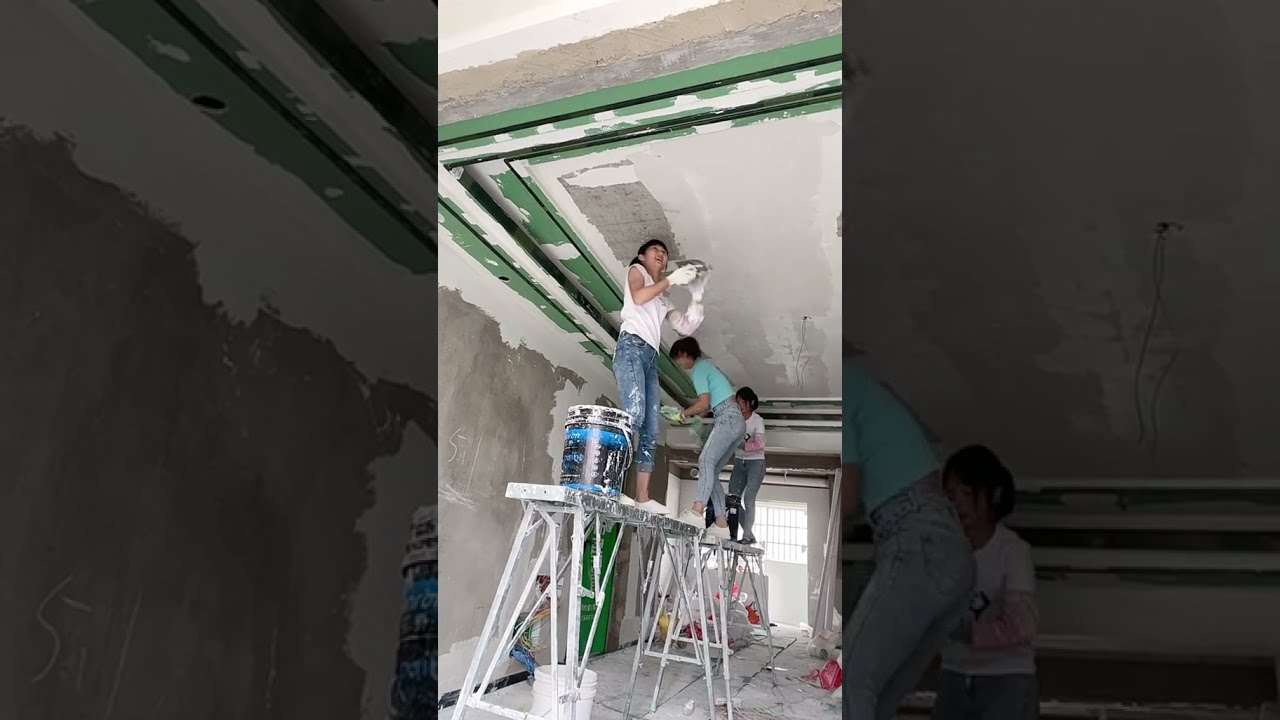This indoor photograph captures three young women, possibly teenagers, engaged in painting the ceiling of what appears to be a well-decorated room within a house. They are precariously positioned on a tall, silver scaffolding splattered with paint. All three wear tight blue jeans, and their shirts vary in color: two in white (one of these is sleeveless, the other has pink sleeves) and one in a vibrant lime green. They are all of Asian descent, with paint noticeably on their hands and clothing, further emphasizing their hands-on involvement. The ceiling they are painting appears intricate and partially decorated in green, hinting at a plaster finish on what seems to be a concrete structure. Surrounding their work area are large buckets and other painting equipment. Some parts of the image are enlarged and darkened, used creatively as border frames that reveal more details of the unpainted wall and the women working. Overall, the scene encapsulates a vivid moment of teamwork and effort amidst an ongoing home improvement project.